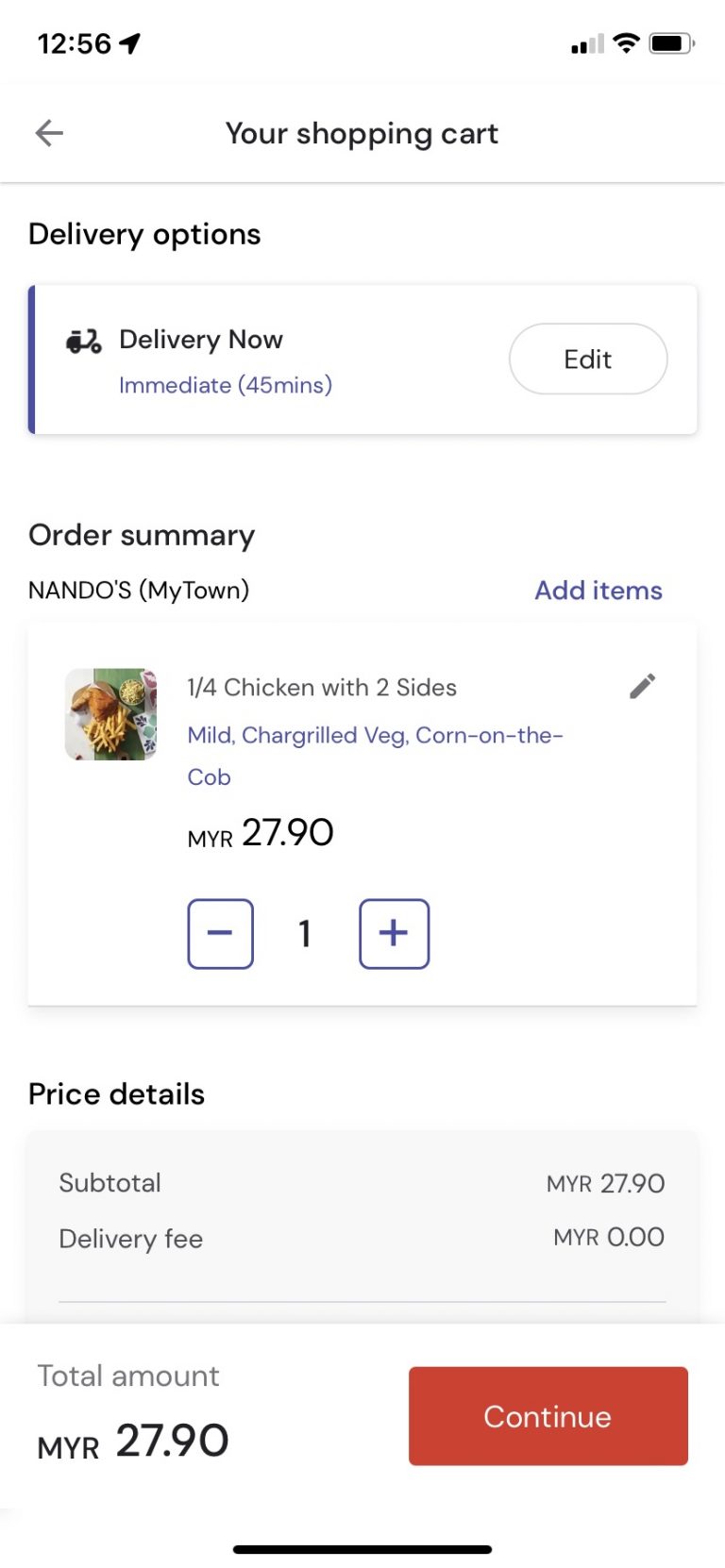This image captures a screenshot of a shopping cart interface on a mobile phone. At the top, there is an arrow pointing to the left, leading the eye to the text reading "Your Shopping Cart". Just below, under the "Delivery Options" section, the delivery mode is set to "Deliver Now (Immediate 45 minutes)," with an "Edit" button positioned next to it for potential modifications. 

Following the delivery options is the "Order Summary" section, which lists the restaurant as "Nando's My Town". Here, the phrase "Add Items" prompts the user to include additional items in their order. The current selection displays "1/4 Chicken with Two Sides: Mild Char-grilled Veg, Corn on the Cob," priced at $27.90. There is a quantity adjustment feature with a minus sign in a box on the left and a plus sign on the right, allowing the user to modify the number of items ordered.

Further down, the section labeled "Price Details" breaks down the costs. The subtotal is listed as $27.90, with the delivery fee marked as free (MYR 0.00), bringing the total amount to MYR 27.90. At the bottom of this section, there is a prominent red "Continue" button, guiding the user to proceed with the order.